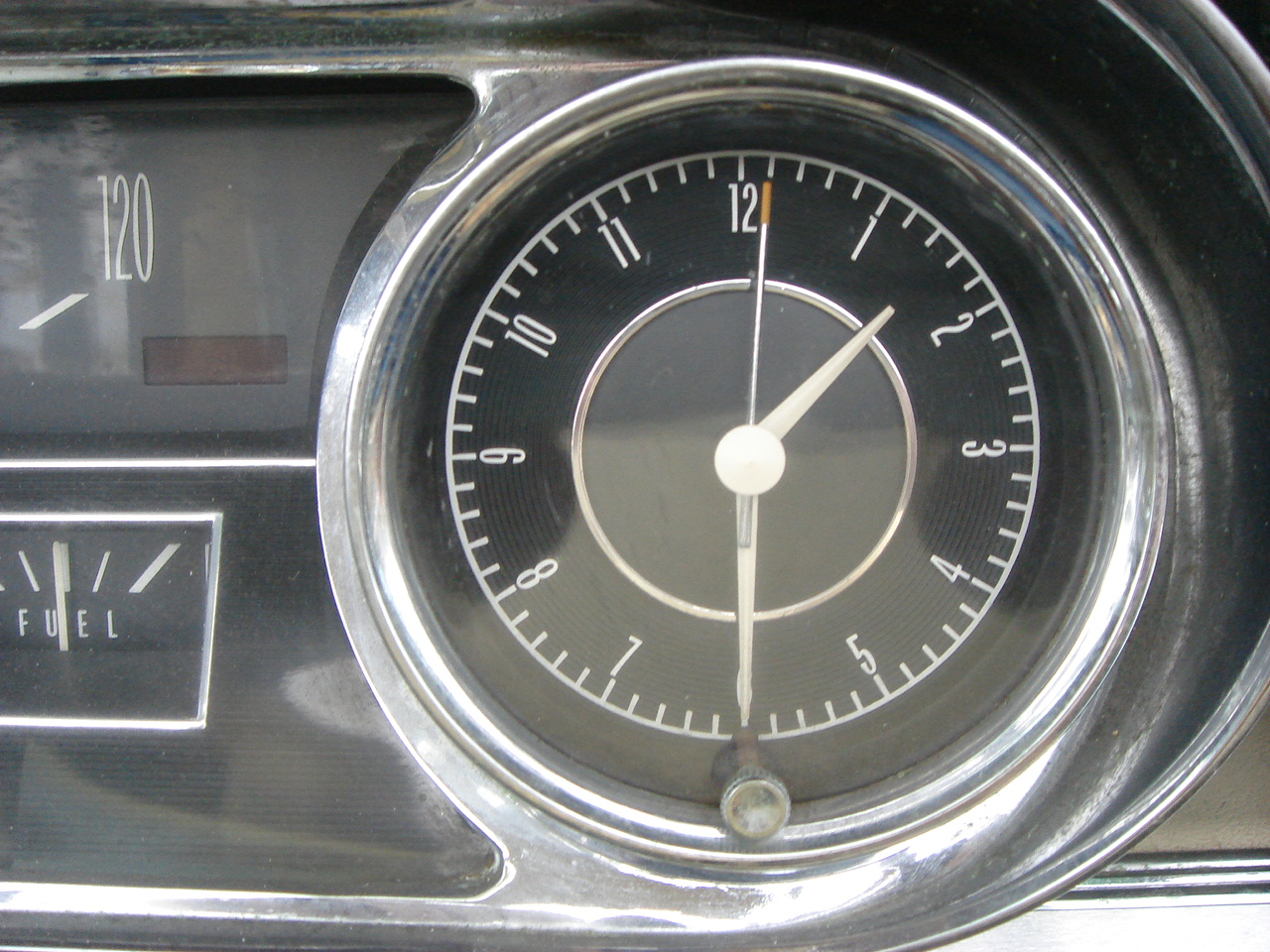This close-up photograph captures the intricate details of a car's dashboard clock, framed in a polished silver chrome bezel. At the heart of the clock, the face is a dark black circle, featuring a small central white circle outlined by a gray ring, which is further bordered by a slim line of silver. Encircling this central design, the outer edge is marked with a white ring filled with minute indicators represented as dashed lines. The hours are denoted with bold white numerals, and the hour and minute hands are similarly white, while the second hand is distinguished by a red tip.

To the left of the clock, the edge of the car's speedometer is visible, featuring a diagonal white line set against a black background, with the number '120' displayed prominently in white above it. Below this, there’s a small red rectangular indicator. Continuing downward, a silver chrome line separates the speedometer from the adjacent fuel gauge. The fuel gauge itself is outlined in thick white and labeled with 'Fuel' in white letters. Vertical and angled lines within the gauge indicate the fuel level. This detailed image captures the sophisticated and functional aesthetic of the car's instrumentation.